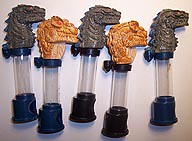This image features five small, cylindrical containers, each mounted on a clear tube with a distinct dinosaur or dragon head design. Arranged against a white background, the heads alternate between dark grey and a yellow-orange hue, with varying details that suggest some may have red eyes. The bases of the tubes appear to be either black or blue, depending on the creature coloration. The intricacy of the carved heads, which resemble prehistoric creatures, suggests they may be promotional items for a show or movie. The picture's limited resolution makes it challenging to discern the exact material of the tubes and bases, but they resemble plastic or metal elements.